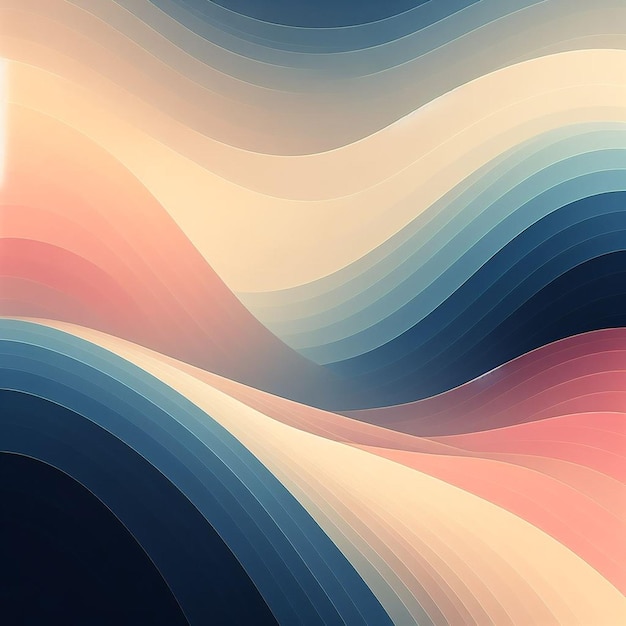The image is an abstract painting featuring a series of flowing, wave-like lines reminiscent of ribbons or a flag waving in the air. At the top, the lines start with a gradient of blues, transitioning from dark blue to light blue, and eventually blending into white. This sequence repeats, with the blues becoming darker towards the lower left-hand corner, which almost appears black. Alongside the blue hues, the painting features pink and dark pink waves, as well as shades of tan, cream, peach, and gold. These colors interweave in a harmonious pattern, creating a dynamic composition of light and dark that captures the fluidity and motion of the abstract design.